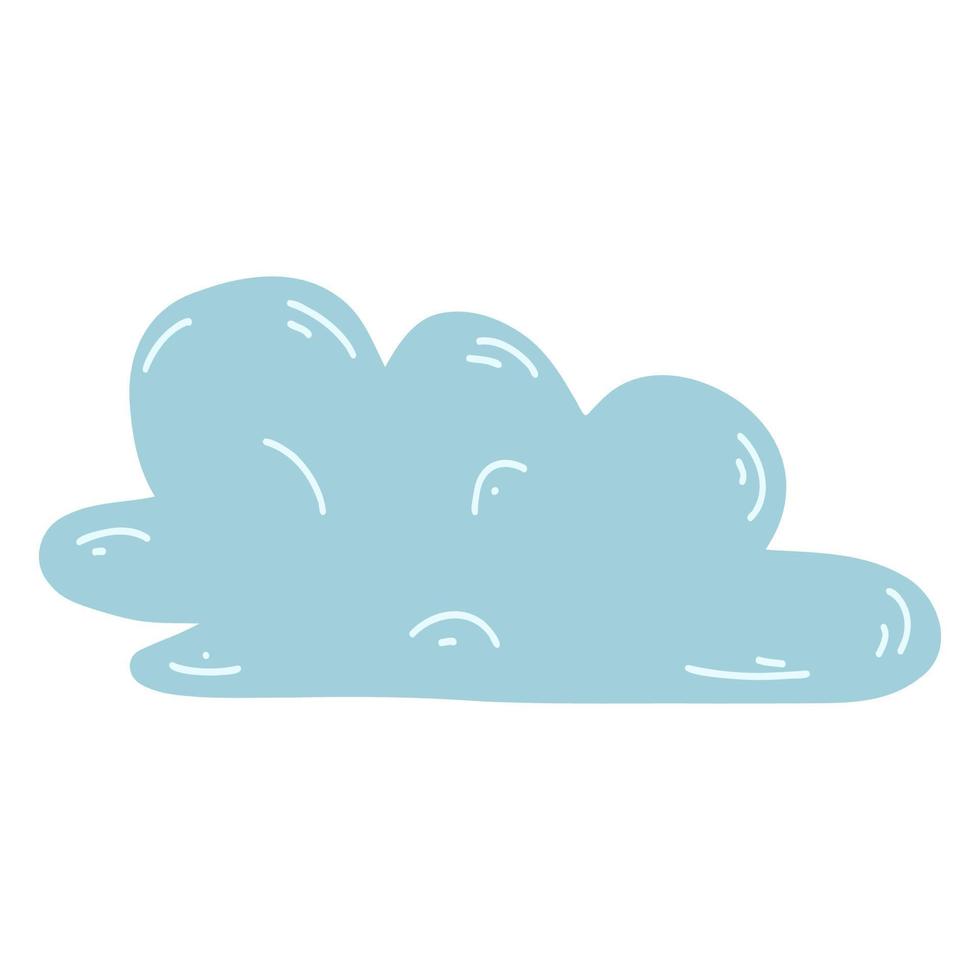The image is a color illustration of a simple cloud against a white background, characteristic of a child's drawing or that of someone with limited experience. The cloud's shape is somewhat flat on the bottom, while the top is adorned with six rounded humps, more pronounced on the left side. The cloud is primarily a solid aqua or grayish-blue color, giving it a fluffy appearance. To add depth and texture, the illustration includes white curved lines strategically placed along the contours—especially on the top right and left humps and a few on the bottom edges. These highlights contribute to a sense of dimension despite the overall flatness of the drawing.